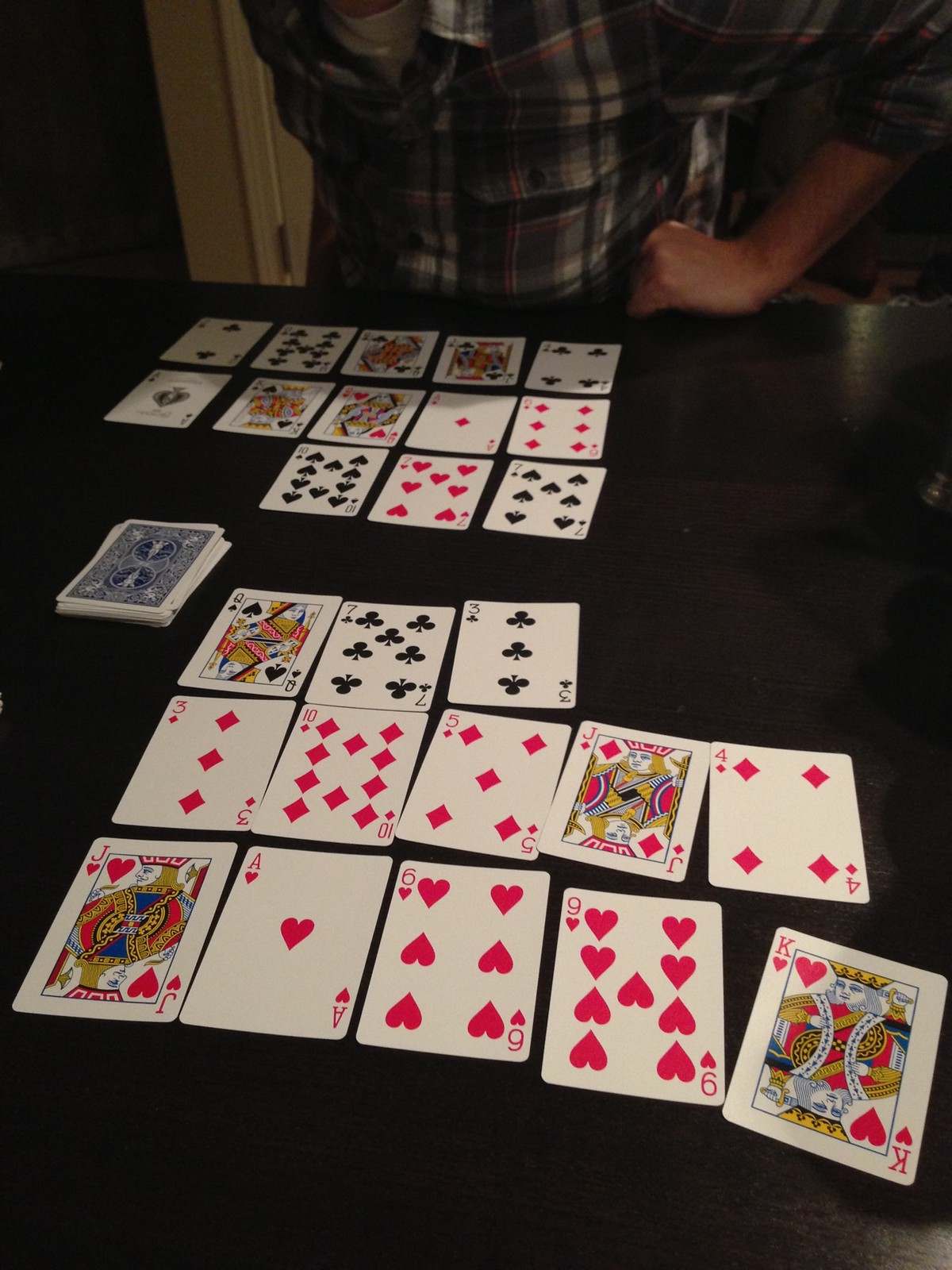In the background of the image, there is an individual wearing a black, white, and red flannel shirt layered over a white undershirt. This person's face is obscured, but their left hand rests visibly on a table. Behind them, part of a white door and its hinge can be seen, contrasting against a tan-colored wall. The scene fades into darkness around these details. 

The main focus of the picture is a dark wooden table adorned with several playing cards. In the back by the person, there are 13 cards spread out. A stack of cards with blue backs occupies the middle left section of the table. In the foreground, another 13 cards come into view. From back to front, the visible cards are a 2, 10, queen, jack, 4, ace, king, queen, ace, 6, 10, 7, and 7. The cards closest to the front include a queen, 7, 3, 3, 10, 5, jack, 4, jack, ace, 6, 9, and king.